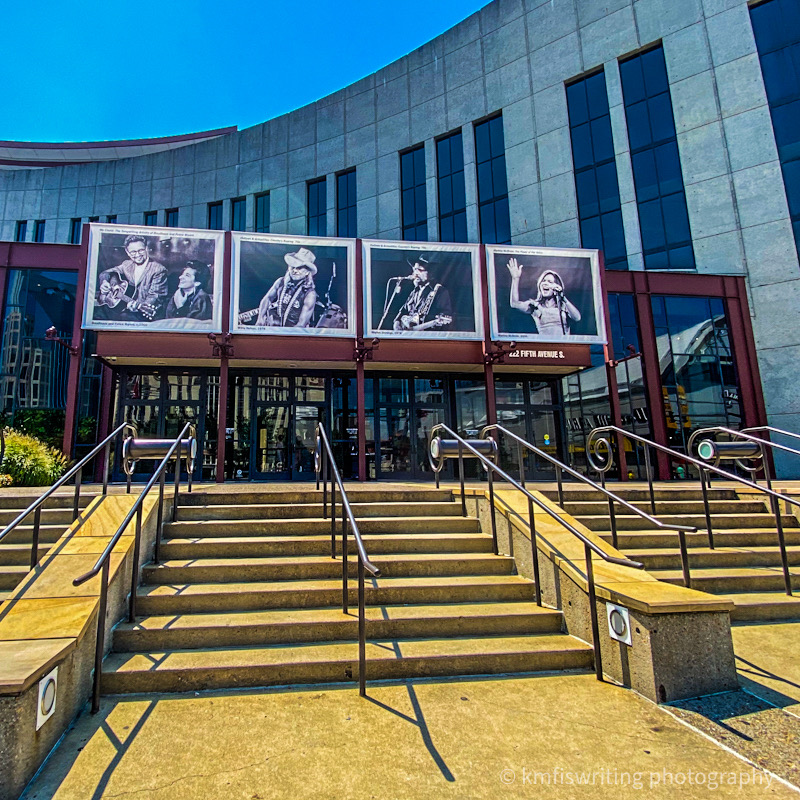This image captures the exterior of a large, predominantly gray concrete music hall, possibly located at 222 Fifth Avenue in New York. The massive building, with its curved facade, features tall, narrow glass windows arranged both vertically and horizontally at the front. The entrance is marked by a red border displaying black and white photographs of notable country and western artists, including possible appearances by Johnny Cash and Willie Nelson. 

The outdoor stairwell leading up to the multiple doorways is paved with concrete and includes handrails, some styled like music notes, adding to the artistic theme of the venue. A small sign near one of the doors reads "Lafoyer" and hints at the main auditorium inside. At the bottom-right corner of the image, there is a watermark indicating "KMFIS Writing Photography," crediting the photographer. Above the entire scene is a clear blue sky, providing a picturesque backdrop to this iconic music venue.